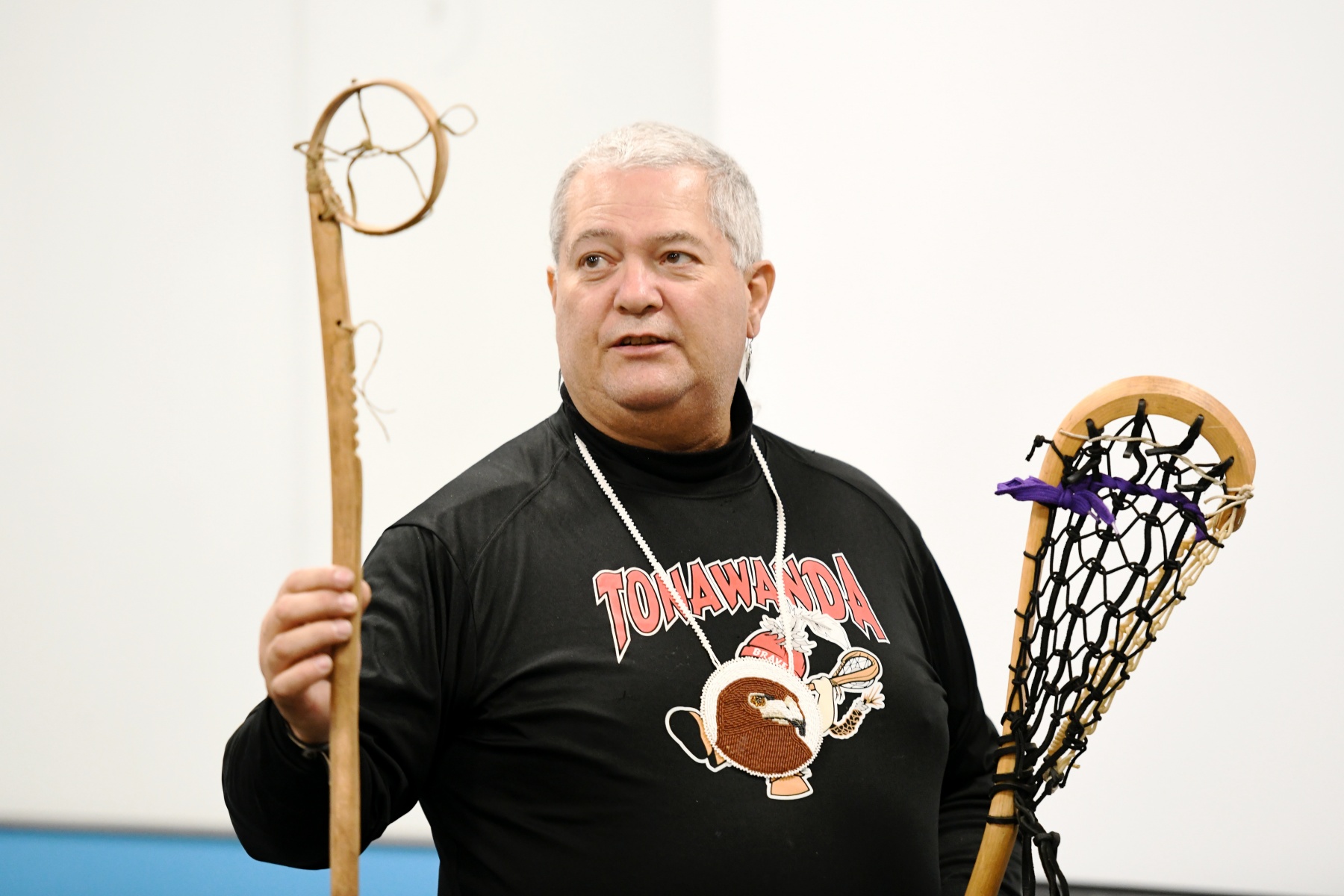The image depicts an older, somewhat overweight man with short white hair, possibly in his 60s. He has an earring in his left ear and is wearing a black long-sleeve turtleneck shirt featuring the text "Tonawanda" in red text outlined in black and white. The shirt displays an artwork of a cartoon figure holding a lacrosse stick, partially covered by a round pendant hanging from a white rope around the man's neck. The pendant showcases a brown bird, possibly a hawk, with a white face and a black-tipped beak. The man is holding two lacrosse sticks: one in his left hand is a modern wooden lacrosse stick with black and purple threads, and the other in his right hand is a more traditional, ancient-looking lacrosse stick with a simple circular head, reflecting its indigenous origins.